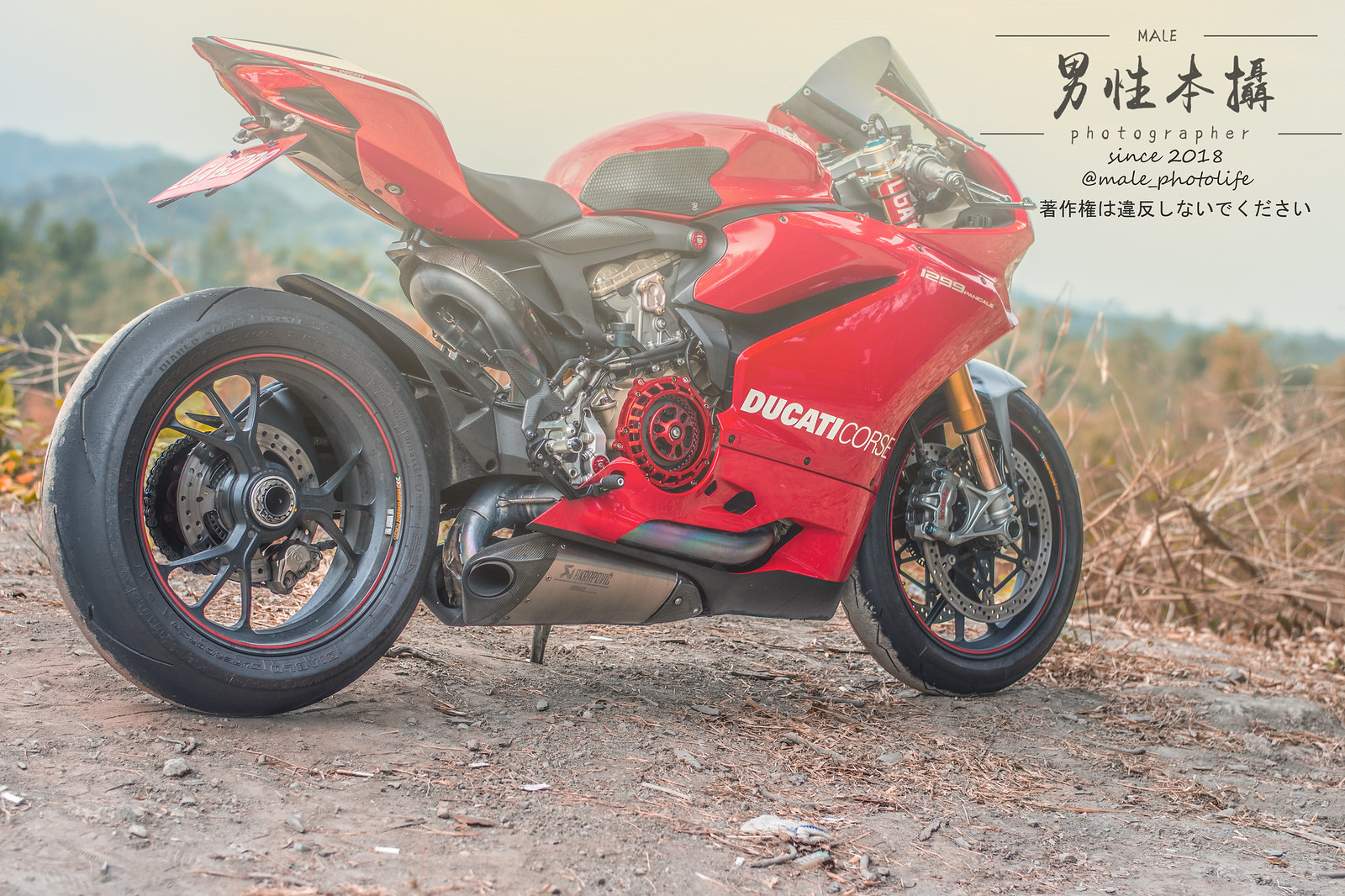This photograph showcases a Ducati Corse motorcycle, prominently displayed as if for an advertisement. The motorcycle is positioned on a grayish dirt road, surrounded by a natural backdrop featuring a brownish grassy hill, green trees, and a distant mountain, all beneath a gray sky. The bright, shiny red chassis, seat, and main body of the motorcycle are strikingly contrasted by its black tires and gray metal spoked wheels. The bike faces to the right, resting on its kickstand. 

In the upper right corner of the image, black text is visible, providing marketing information. This includes a partially discernible word that may read "H-A-L-E," followed by lines of Asian glyph writing. Below the glyphs, it mentions "since 2018" and an email address "at mail.photo life," flanked by more Asian text. Notably, the right side of the motorcycle features the distinct white lettering "Ducati Corse," enhancing its identity as a high-end, stylish vehicle.